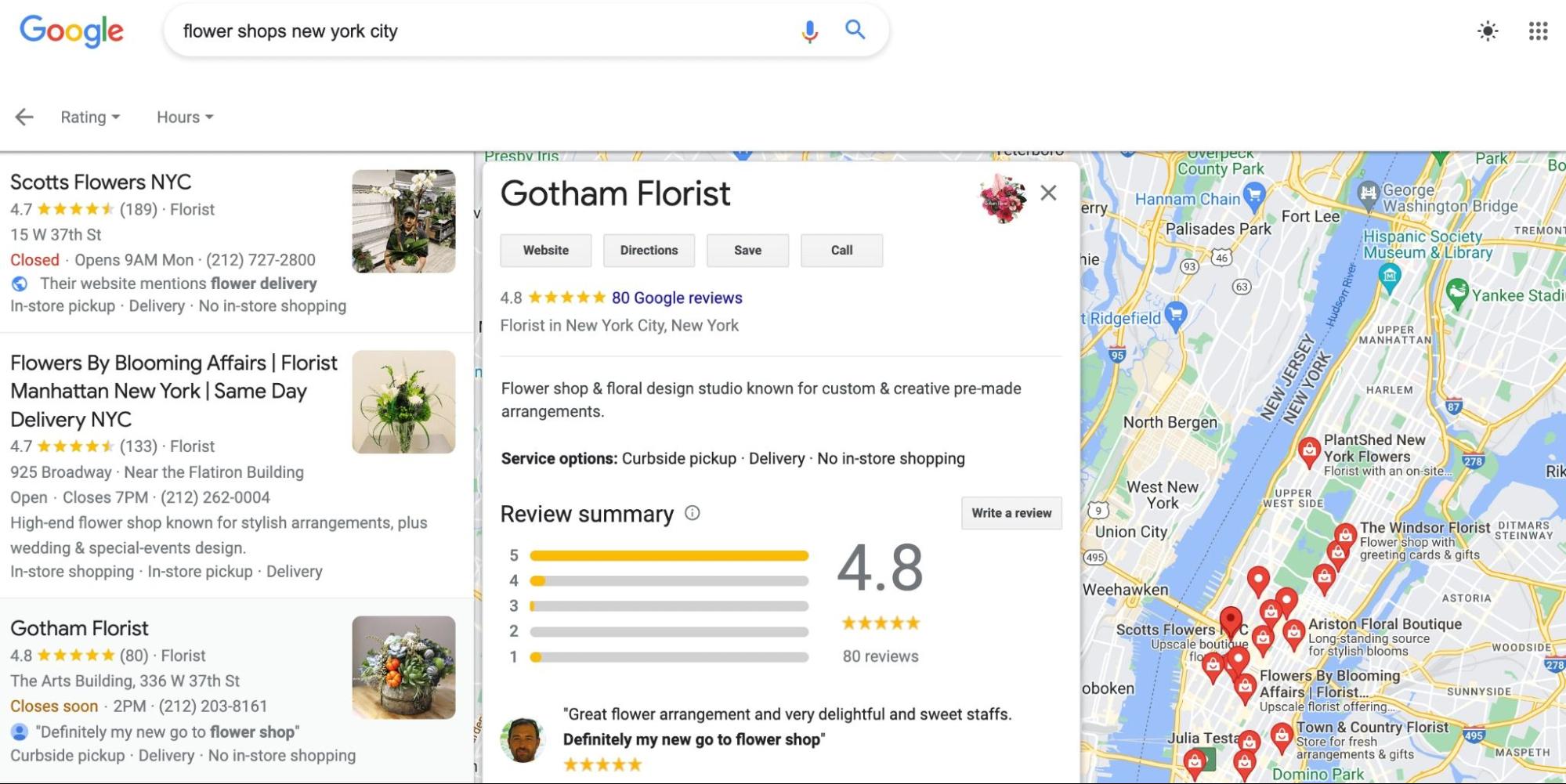**Detailed Caption:**

The image is a screenshot from Google displaying search results for "flower shops New York City." The Google logo at the top features its traditional colors: blue, red, yellow, blue, green, and red. Beneath the search bar containing the phrase "flower shops New York City," three prominent flower shops are listed along with their ratings and hours of operation.

1. **Scott's Flowers New York City** appears first, boasting a 4.7 out of 5 rating.
2. **Flowers by Blooming Affairs - Florist Manhattan New York City** follows, also with a 4.7 rating and notes that they offer same-day delivery.
3. **Gotham Florist** is listed last with a higher rating of 4.8 based on 80 reviews. It indicates that they will close soon at 2 p.m. A highlighted customer review mentions, "Definitely my go-to flower shop." This listing has been clicked to open for more detailed information.

A map situated on the right reveals numerous flower shops in the New York City area. The Gotham Florist listing features their logo, which incorporates floral imagery. Options to visit their website, get directions, save the listing, or call the shop are clearly available. Beneath, customer reviews and additional details about the florist are provided. The searcher has ample choices for purchasing flowers in New York City.